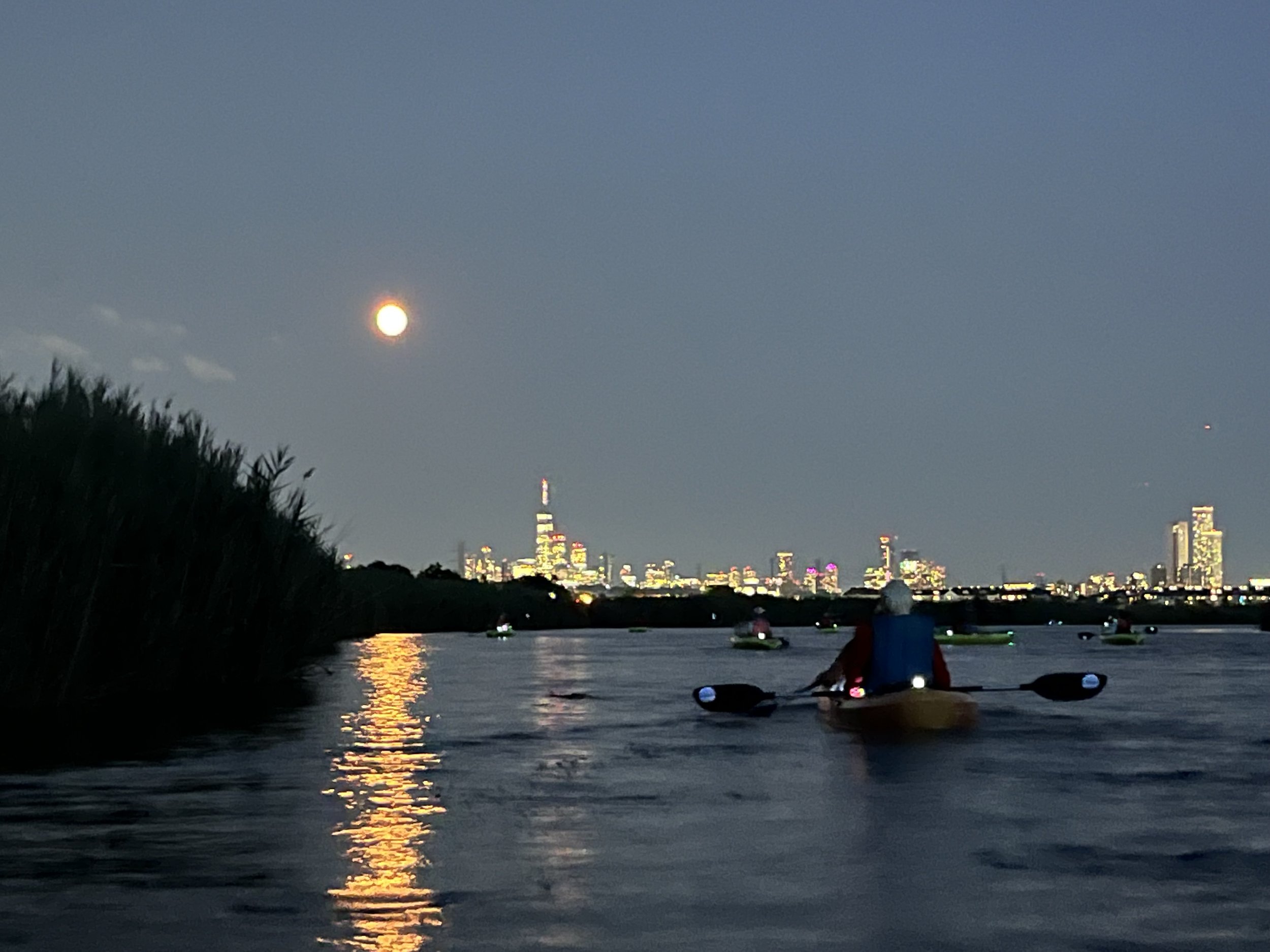This nighttime photograph captures a serene scene of a bay illuminated by the soft glow of a nearly full moon and the vibrant lights of an expansive city skyline on the horizon. The sky, a muted gray-blue, is brightened by both the moon and the illuminated skyscrapers and smaller buildings. Reflections of the moon and city lights shimmer across the water's surface, creating a breathtaking visual symphony.

In the foreground, a person in a yellow kayak, wearing a blue vest, faces away from the camera, seemingly entranced by the celestial and urban lights. A set of double paddles rests in their hands. Nearby, along the lower right third of the image, other kayakers, some with reflective tape on their backs, add life to the tranquil water. It appears to be a kind of nighttime kayak gathering, with a few of the small, paddle-equipped vessels having tiny lights that dot the scene like fireflies.

The city's lights create a striking contrast with the dark outline of trees and bushy banks extending into the water on the left, enhancing the natural beauty that borders the urban landscape. This blend of nature and city life, punctuated by the quiet activity of the kayakers, creates a harmonious and detailed tableau.